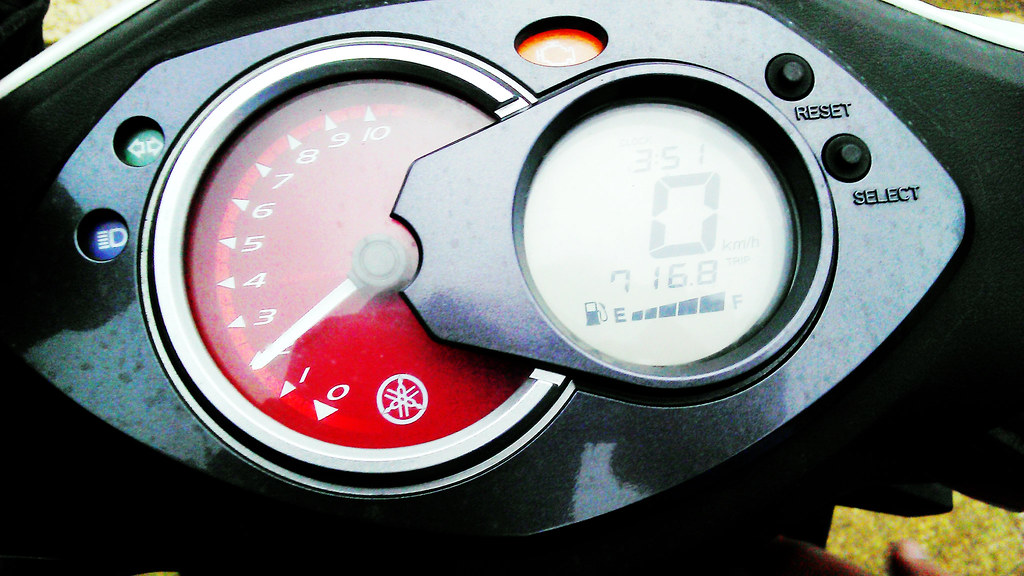This photo features the intricate dashboard of a motorcycle or small engine vehicle, designed in the shape of an almost diamond-like form. The top of the dashboard is flat, while the sides angle outward before curving around and rounding at the bottom.

Dominating the dashboard is a large red analog gauge with a white dial, displaying numbers from zero to ten. Each number is accompanied by a small white triangle that points outward. Beneath this red gauge, a small white round symbol is also visible.

To the bottom right of the red gauge sits a digital display, which overlays it slightly. The digital gauge indicates several metrics: a full gas tank, mileage of 716.8, the time 3:51, and a current speed of zero miles per hour.

Above both gauges, there is a small round orange engine light. Directly to the right of the digital display are two small black buttons, labeled ‘reset’ and ‘select’.

On the left side of the red analog gauge, there is a green blinker button with arrows pointing both left and right, and just below it, a blue headlight button. The detailed layout and color-coded elements of this dashboard provide a comprehensive and accessible display for the rider.